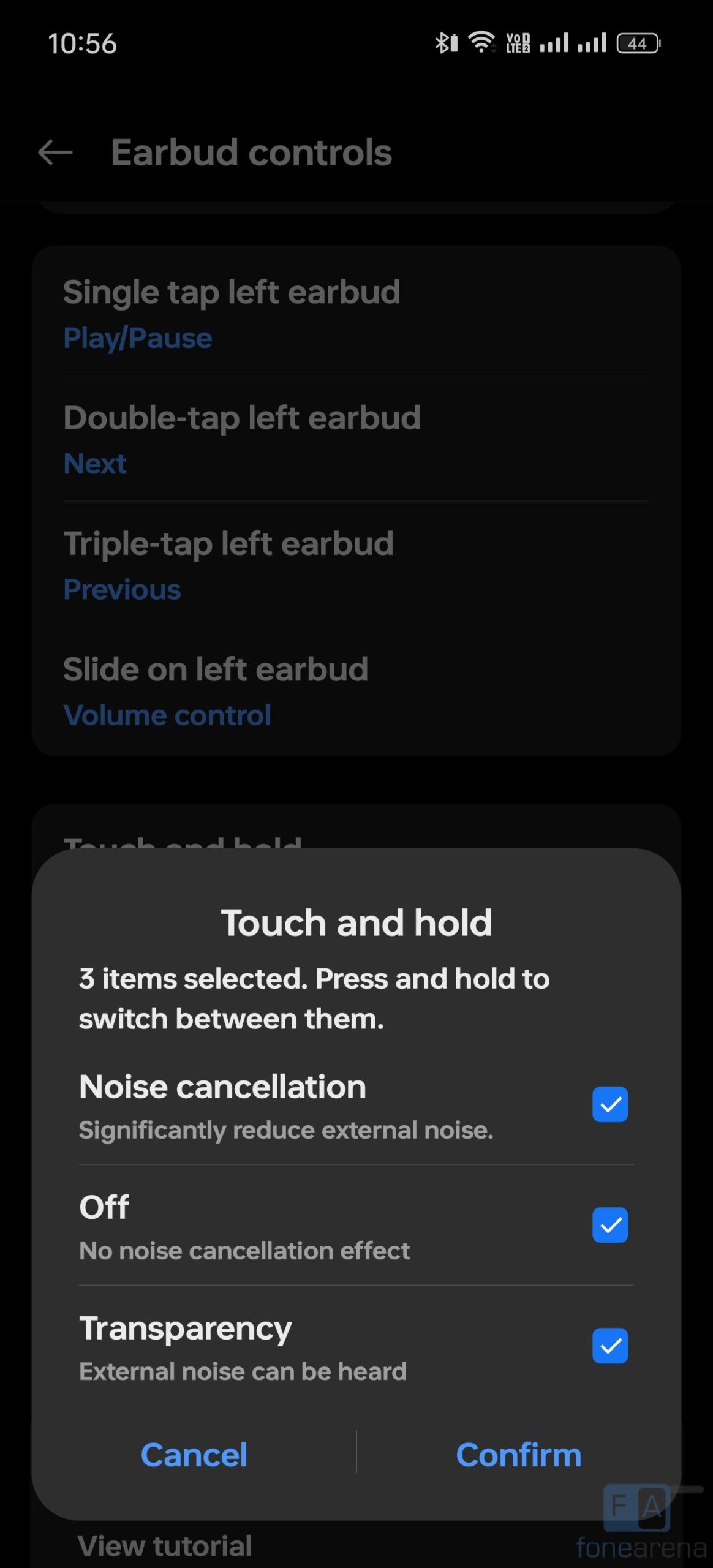This screenshot captures the settings section for earbud controls on a mobile device. At the top, the time is displayed on the left as 10:56, and on the right, you can see icons for battery status, Bluetooth connectivity, and cellular and internet quality. A search bar at the very top reads "Earbud Controls."

The settings are divided into two main sections. The first section details the controls for the left earbud:
- Single Tap: The blue text next to it reads "Play/Pause."
- Double Tap: The blue text indicates "Next."
- Triple Tap: The corresponding blue text says "Previous."
- Slide (left): This option is for volume control.

At the bottom of the screen, there is a pop-up box with rounded corners. The box, with white text, indicates "Touch and hold - 3 items selected. Press and hold to switch between them." The three options listed in this pop-up, each marked with a blue checkmark, are "Noise Cancellation," "Off," and "Transparency." Below these options, there are two buttons labeled "Cancel" and "Confirm."